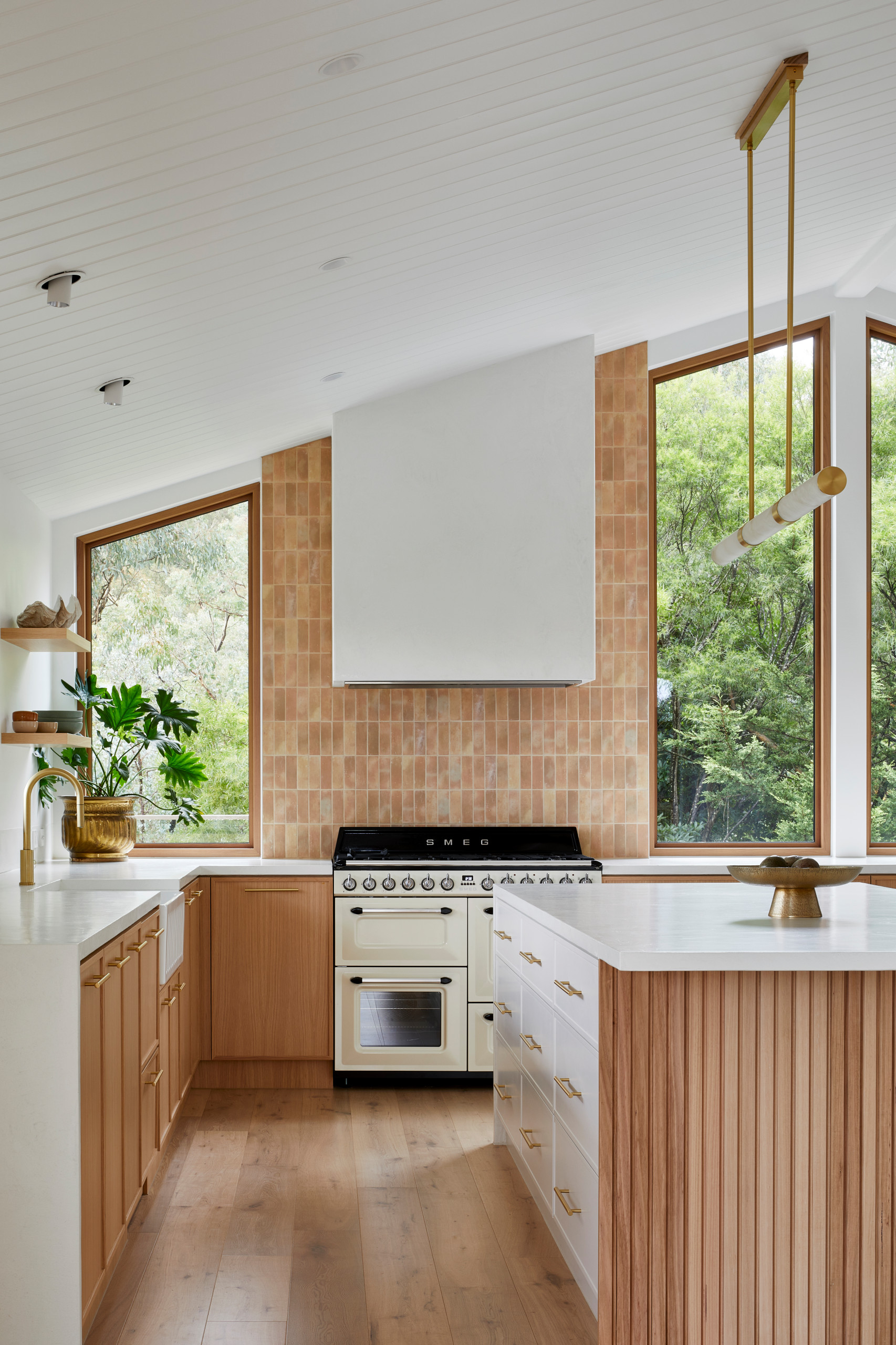In the image, we see a modern, thoughtfully designed kitchen with a distinct, stylish flair, possibly suitable for an architectural magazine. The kitchen features a prominent right-side island equipped with nine white drawers adorned with gold handles. The island boasts a white countertop and its sides are lined with thin vertical strips of light to medium-colored wood. An intriguing sloped, white ceiling peaks at the island's right side, from which multiple lights hang, including a noteworthy bronze hanging lamp attached to two metal poles that support a long cylinder of white with bronze accents. 

The kitchen floor is covered in elegant wood tile, visible prominently in the lower left part of the image. The area also includes additional white countertops along the far left, paired this time with brown drawers and cabinets, consistent with the kitchen's white and brown color scheme. Two trapezoid-shaped windows of varying heights sit on the middle wall with a brick stone wall between them, adding a rustic touch. Below the windows, a stainless steel SMEG oven and stove are centrally featured—though described variably, it stands out with a black top and multiple doors, underscoring its importance in the kitchen.

Amidst the clean, minimalist decor, a bowl filled with fruit sits on the right-side counter, contributing a splash of color. Additional details include plants and the visibility of the sink area on the left, emphasizing the kitchen's practicality and design coherence.